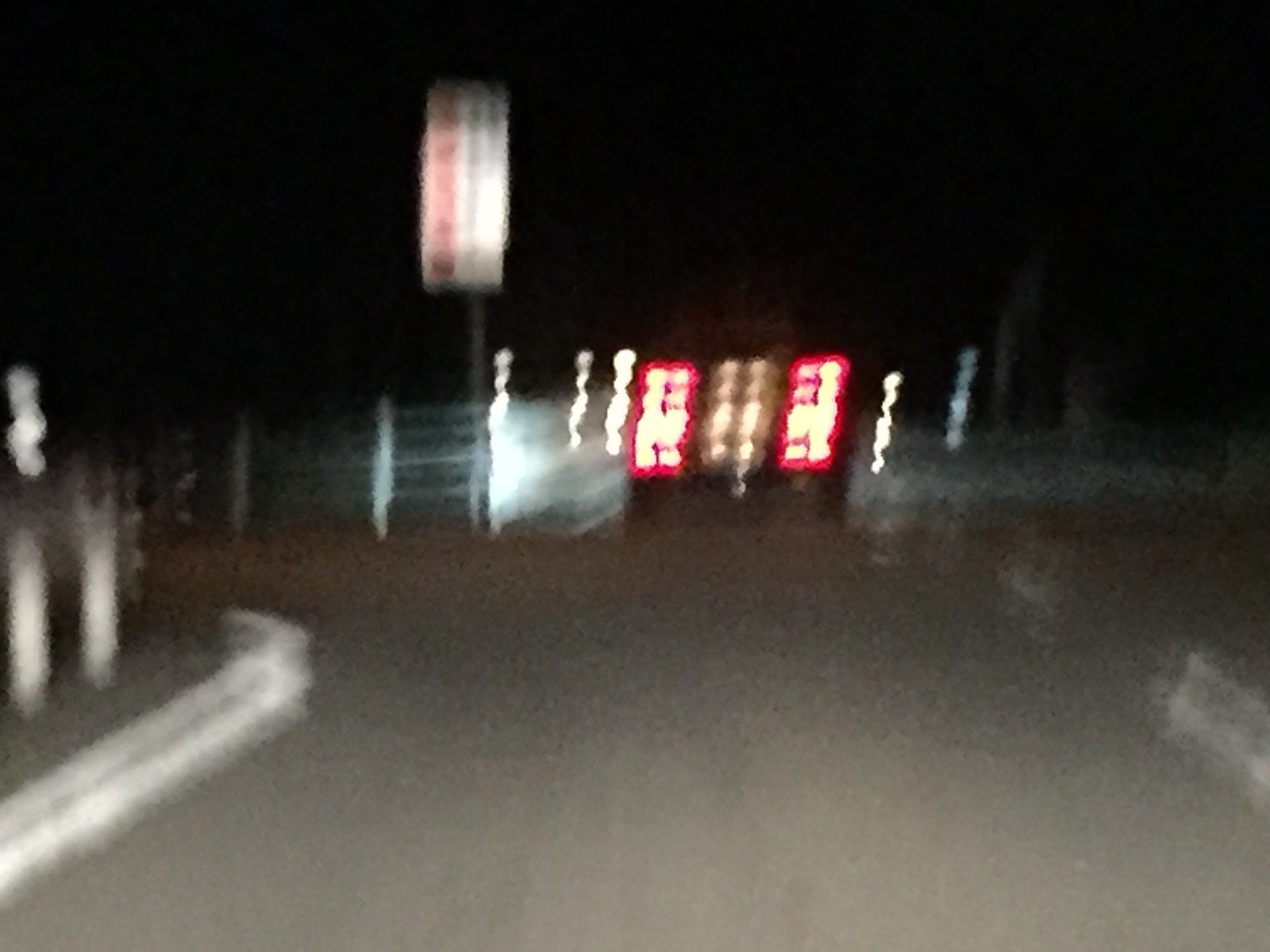This nighttime image captures a blurry street intersection, featuring a prominent curb and a grassy area on the left side. The opposite side of the street is lined with a horizontal metal fence that merges vertically along the sidewalk. A lone car is positioned in the center, traveling straight away from the camera, with its distinctive red brake lights and yellow lights in the midsection clearly visible. Adding to the scene's visual confusion, a white sign with indecipherable red and black writing stands elevated on a pole. The background suggests possible tree branches and maybe snow, although the extreme blurriness makes details hard to confirm, contributing to an overall sense of distortion and uncertainty.